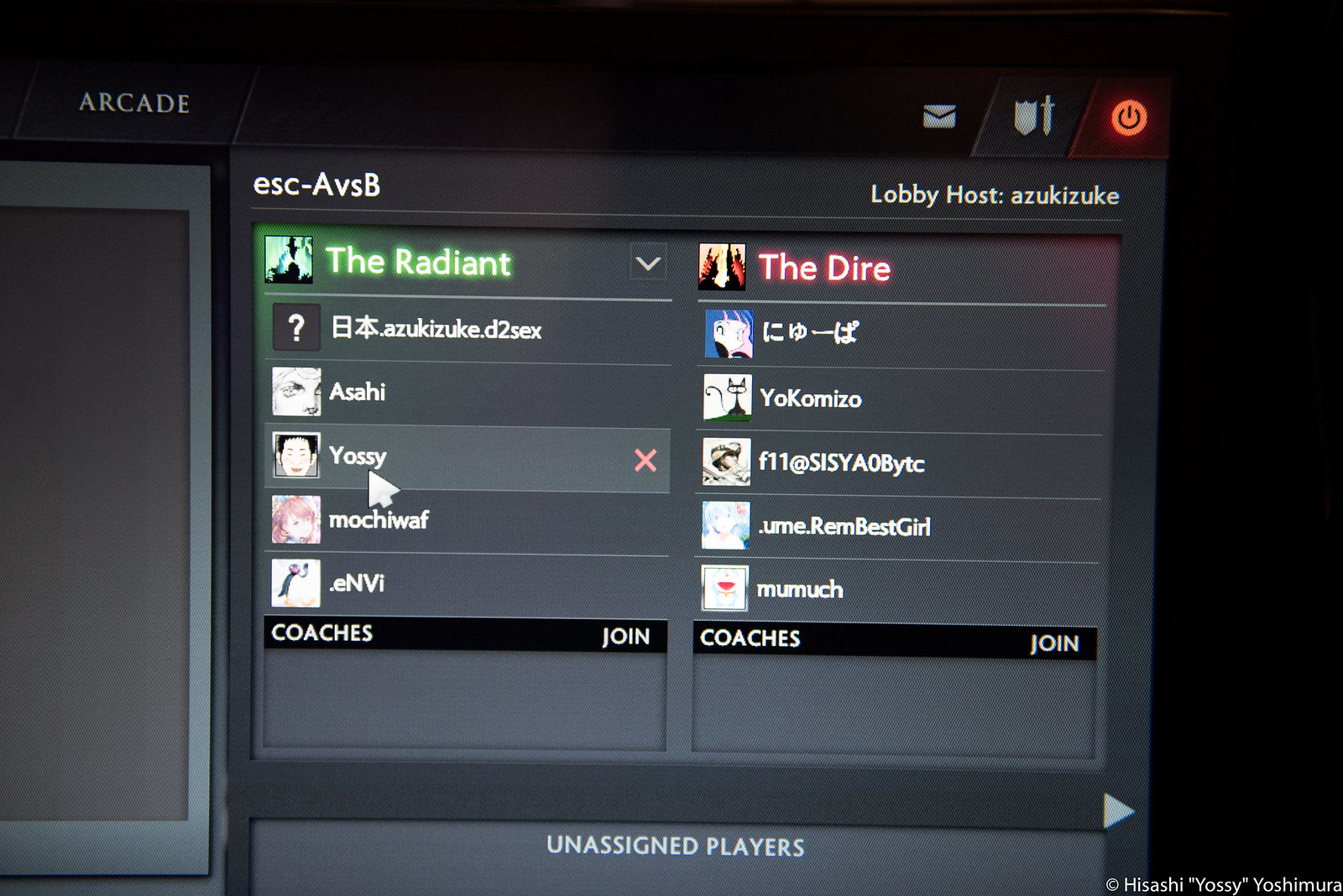The image depicts a detailed screen from a video game lobby styled like an arcade. At the top of the screen, the word "ARCADE" is prominently displayed in white text in the upper left-hand corner. Adjacent to this, on the right, is a red power button. The game menu is divided into multiple sections: in the middle, two lists labeled "The Radiant" in bright green and "The Dire" in pink are visible, each containing five player names paired with small head icons as identifiers. Although the names are not clearly legible, one name in each list is marked with a red X, indicating the option to delete or deselect the player. Surrounding these lists are various icons, including an email symbol and a sword-and-shield emblem. Further options such as "Coaches" and "Join" are highlighted in black rectangles with white text, followed by a section labeled "Unassigned Players" at the bottom in light gray, all in capital letters. The screen's color scheme features a mix of black, gray, white, pink, green, red, and blue elements, creating a vibrant and organized interface typical of a competitive gaming environment.